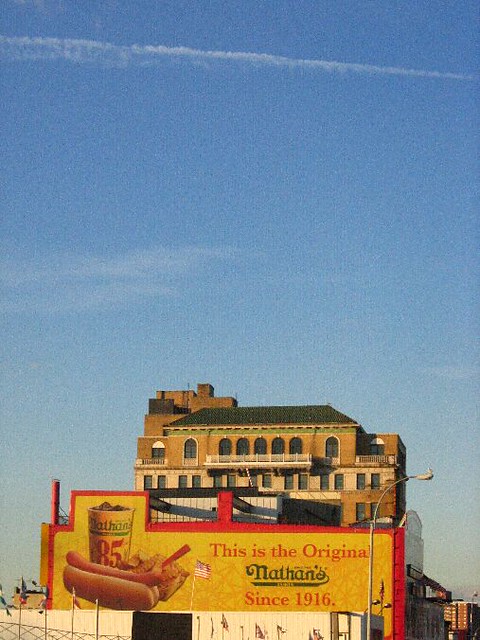A captivating cityscape under a stunning blue sky with a prominent contrail streaking from the left to the right, suggesting the recent passage of an airplane. Scattered wispy clouds dot the skyline, adding to its charm. Dominating the scene is an older brick building, characterized by its intricate architectural details. The top floor boasts arched windows, and the roof appears to be made of slate. The building's facade is a patchwork of brick shades: lighter bricks adorn one floor, while the rest of the structure features a rich yellowy-red brick. Along the side of the building, there's a vibrant painted billboard advertising Nathan’s Hot Dogs. The classic advertisement features a red border and a bright yellow background with text declaring "This is the Original Nathan's Since 1916." It showcases a mouthwatering hot dog in a bun, a paper cup filled with iced soda prominently branded with "Nathan's" and "85," a cardboard tray of golden French fries with a small fork, and an endearing touch—a tiny American flag planted in the fries. This image captures both the charm of urban architecture and the nostalgic allure of a beloved American eatery.